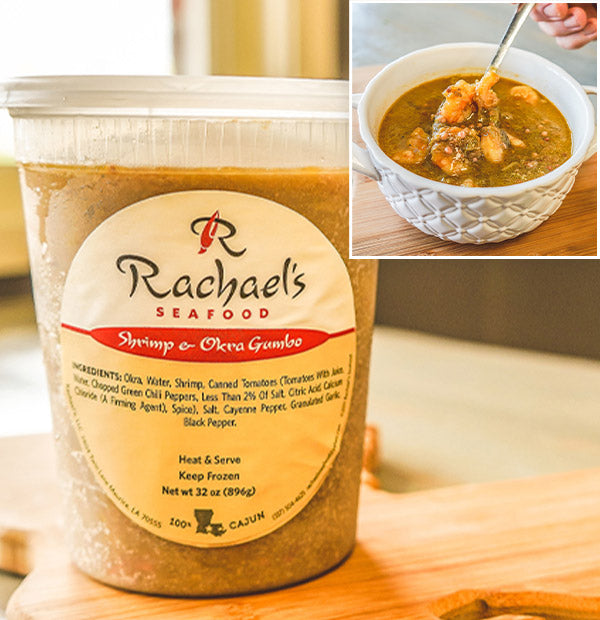The image prominently features two components. The larger section, roughly 70% of the image, showcases a clear plastic takeout container labeled "Rachel's Seafood, Shrimp and Okra Gumbo." The label is detailed with ingredients including okra, water, shrimp, canned tomatoes, chopped green chili peppers, less than 2% salt, citric acid, calcium chloride, firming agent, spices, cayenne pepper, granulated garlic, and black pepper. Additional label information includes instructions to "heat and serve" and "keep frozen," a net weight of 32 ounces (896 grams), and a note that it is "100% Cajun." The logo features a script R, where the vertical line is a chili pepper. 

On the upper right corner of the image, an inset shows a close-up view of the gumbo served in a white ceramic mug with two handles. The gumbo, rich with visible shrimp and okra, is being scooped out with a spoon, ready for serving.